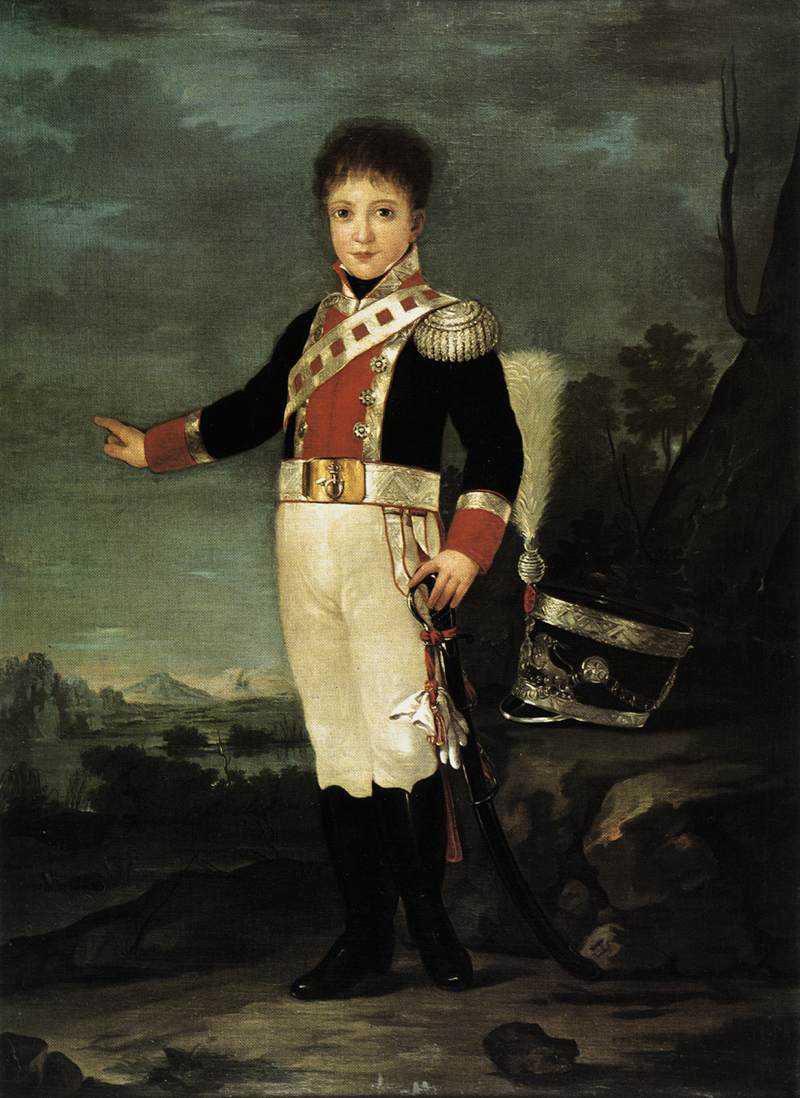This detailed painting features a young boy standing outdoors on a rocky surface, set against a backdrop of cloudy skies, distant waters, and mountains. The boy, with light skin and dark brown hair, is dressed in an elaborate military uniform reminiscent of the Napoleonic era. His uniform includes a black jacket with a red center and cuffs, outlined in gold, gold shoulder pads, and a gold and red sash across his chest. He dons white breeches and knee-high black boots. The boy's right arm is extended and pointing towards the left of the frame, while his left hand rests on the hilt of a sword. His expression is direct, as he looks forward at the viewer with round doe eyes and small pouty lips. To his right, on a piece of stone, lies his tall black hat, adorned with silver braiding and a prominent white feather. The colors in the painting range from black, gray, and tan to off-white, red, silver, and gold, contributing to the dramatic and historical atmosphere.